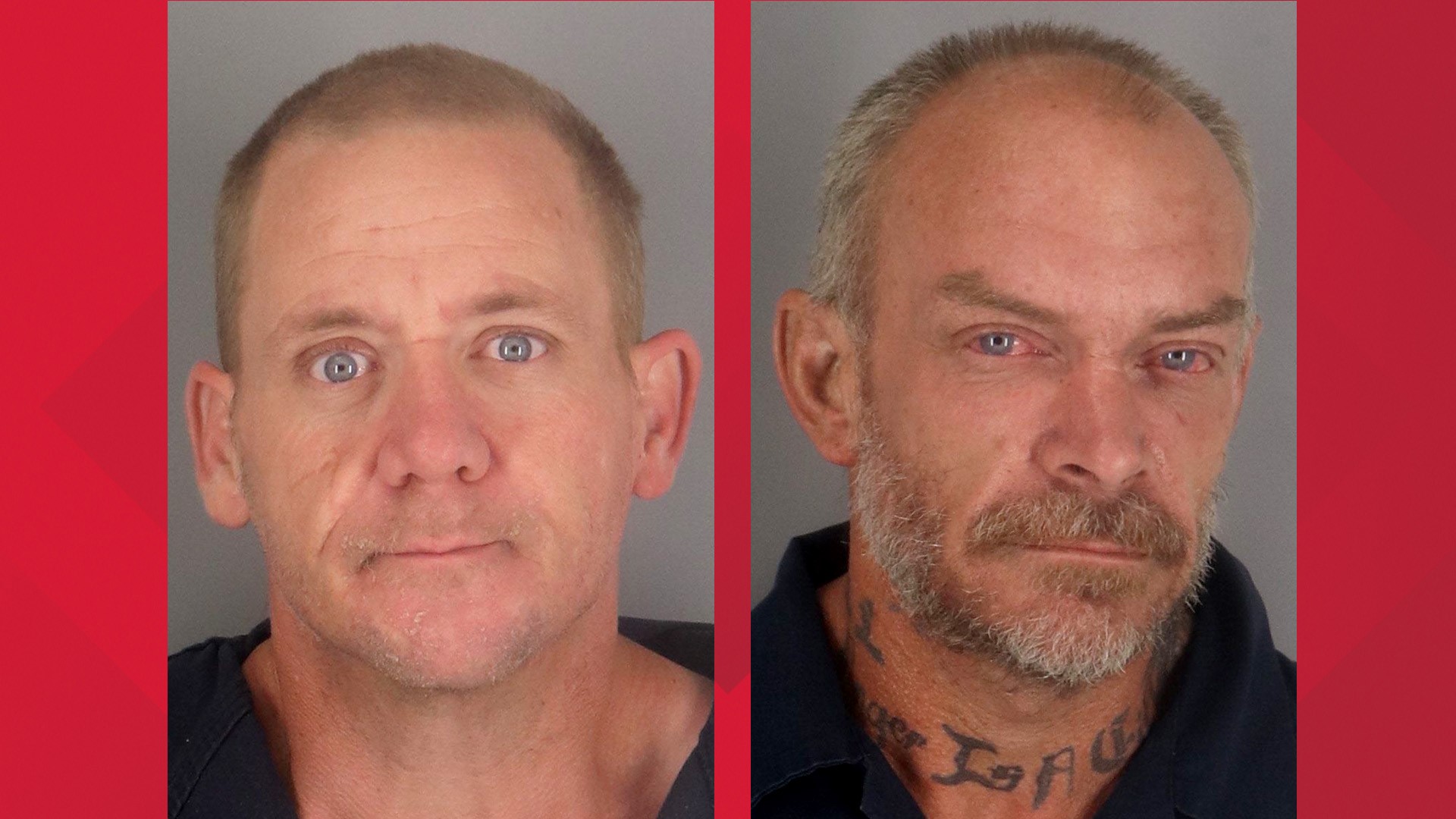The image features two mug shot-style photographs against a striking bright red background. The man in the left photograph has a close-cropped, dirty blonde buzz cut and vivid blue eyes. His face shows some wrinkles across his forehead, his nose is thick and meaty, and his left ear appears protruded and slightly red. He has a neutral expression and is wearing a black shirt or jacket, though only his face and neck are visible.

Separated by a thin red line, the photograph on the right depicts another white man with a receding hairline and salt-and-pepper hair. His blue eyes appear bloodshot, and he sports a salt-and-pepper mustache along with a bit of a goatee. He has a slight smirk on his face and wears a black garment. Notable are the thick, black tattoos with unreadable wording that adorn his neck. Both men stare directly into the camera, capturing the viewer's attention with their distinct, rugged looks.